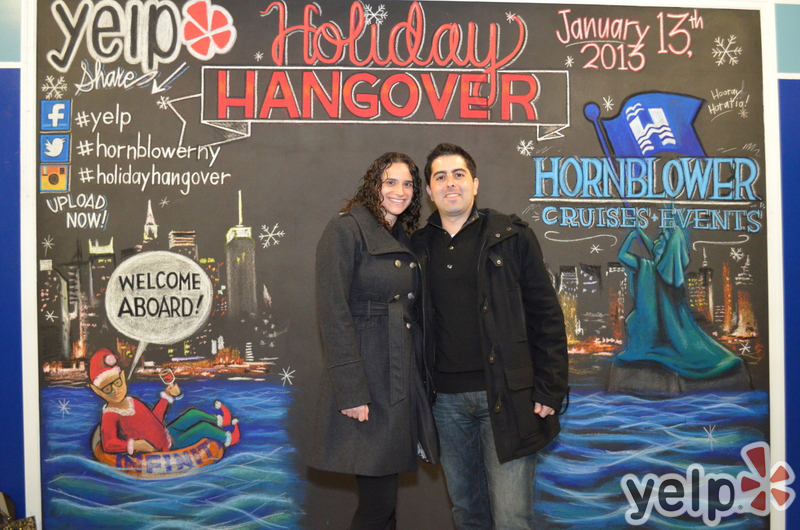A couple in their 30s or 40s are posing in front of an event billboard, both smiling with their arms around each other's shoulders or lower backs. The man, dressed in a black jacket and jeans, and the woman, in a gray jacket and pants, stand side by side, looking directly at the camera. Behind them, the billboard is decorated with drawings of snowflakes and prominently features the text "Holiday Hangover" in red, alongside the event date "January 13, 2013." It also mentions "Hornblower Cruises and Events," with logos for Yelp, Facebook, Twitter, and Snapchat appearing in various corners of the image, encouraging viewers to "Upload Now." The backdrop includes an image of a bay with an elf floating in a life preserver that says "Welcome Aboard," adding a whimsical touch to the scene.